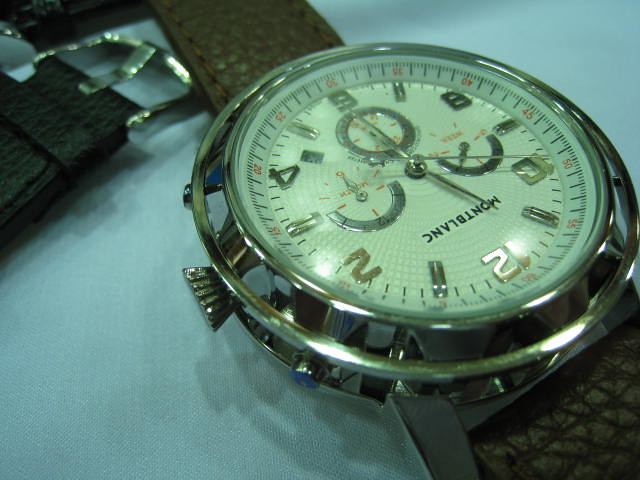This photograph features a close-up view of a wristwatch placed on a teal-blue surface. The watch is positioned slightly off-center towards the right, with its face prominently displayed. The brown leather strap, detailed with stitching along its edges, is partially visible at the lower right and upper left corners of the image. The watch itself has a sophisticated silver-metal bezel and one can see a silver metal winding crown on the left side. Notably, the watch is oriented upside down in the frame, such that the numeral 12 appears in the lower right corner, while the numeral 6 is in the upper left. The face of the watch is protected by glass, underneath which lies a clean white dial. The dial is marked by silver Arabic numerals from 1 through 12, and three sleek, silver hands adorn the center.